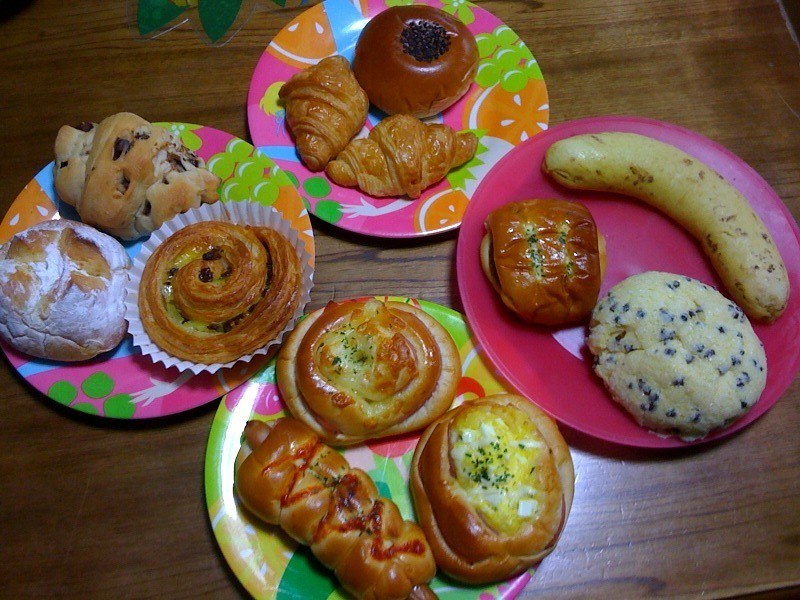This photograph captures a collection of assorted baked goods arranged on a set of four colorful, round plates, all placed on a worn, dinged-up wooden table. The plates are positioned in a diamond orientation, with two at the top and two at the bottom. Each plate features a unique, vibrant design, three of which showcase fruit patterns including oranges and grapes, while one at the three o'clock position is solid pink.

Starting from the top plate and moving clockwise, we observe a spread of pastries beginning with two croissants and a chocolate-glazed donut-like bun. The plate at the three o'clock position, which is solid pink, holds a curved, banana-shaped item, a scone speckled with what might be poppy seeds or blueberries, and a pretzel roll. At the bottom, the plate presents more pretzel rolls alongside another ambiguous pastry resembling rolls with melted butter and chives. The final plate on the left features an array of scones, some dusted with powdered sugar, and what appears to be a cinnamon roll without icing and an apple turnover with black speckles. Each pastry bears a light brown or light yellow hue, interspersed with hints of white flour and butter, adding to the eclectic, tempting display.